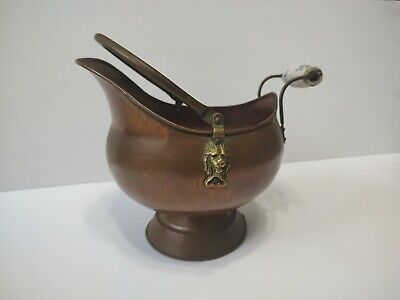This image features an ornate and traditional oriental chamber pot-like vessel, reminiscent of a small pitcher or teapot. The vessel possesses a deep bronze to burgundy lacquer finish, giving it a rich, dark red appearance. It is constructed from a thick, high-quality material that appears to be metal, possibly with wooden elements.

Prominently, there is a decorative gold emblem on the front shaped like a lion, which is a separate, textured piece that can be felt. The vessel has an intricate design including a lip that curves up and to the left, forming a spout-like feature useful for pouring liquids.

On the right side, a porcelain or ceramic handle is attached via a wire that bends and curves upwards. Additionally, there's another longer handle on top that connects to both sides of the vessel, possibly used for carrying. This handle hinges above the lion's head. The vessel stands on a circular base with a ridge just above the bottom, adding stability and elegance.

The scene is set with the vessel placed on a table which casts a light shadow in a grayish environment, positioned near the edge of a wall.